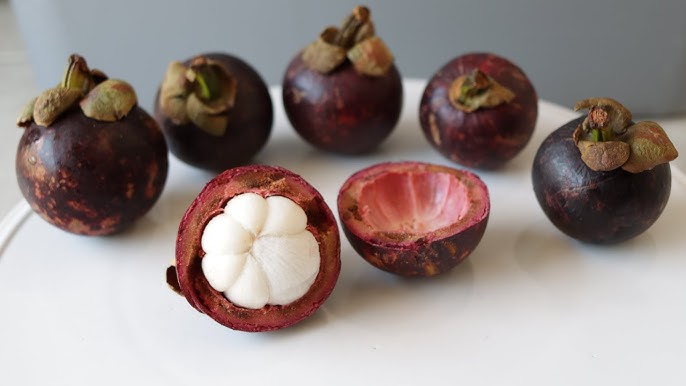This detailed color photograph showcases a neatly arranged composition of nuts. At the forefront, a single cracked nut reveals its segmented white core encased within a reddish-brown shell. This shell is split in half and placed strategically to display both inner and outer textures. Surrounding this central nut are five intact nuts arranged in a linear formation. These nuts boast a rich, dark red exterior, interspersed with lighter red mottling.

Adding a touch of nature, dried green leaves and stems are scattered gracefully atop the ensemble. The entire arrangement rests on a circular white surface, likely a ceramic plate, which contrasts subtly against the muted gray background wall, creating a serene and visually appealing scene.